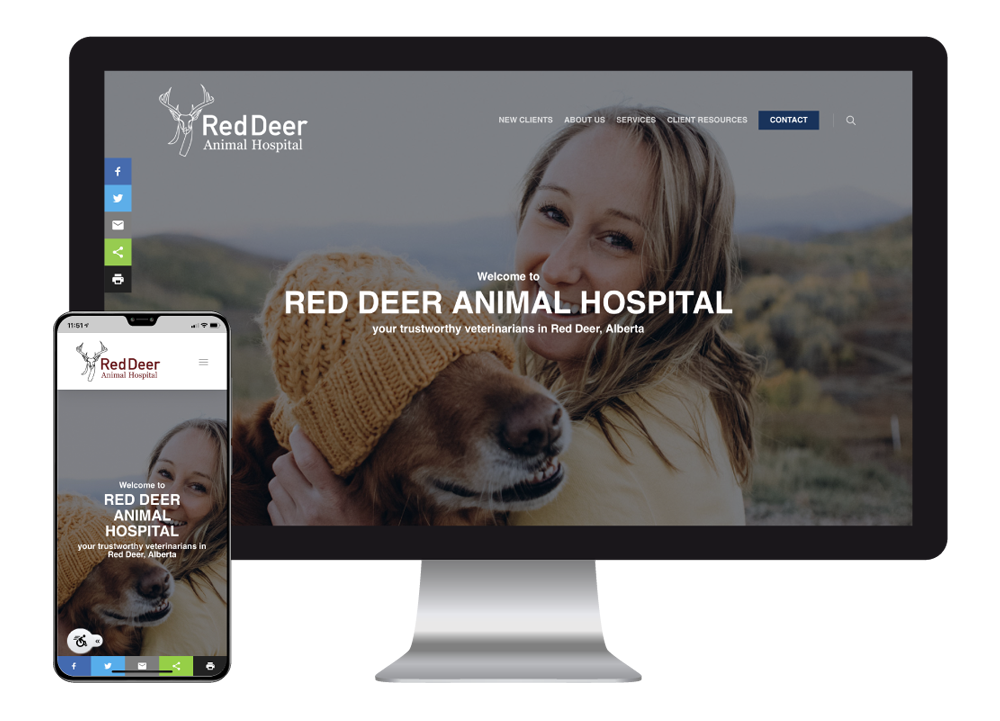The image features a computer monitor with a slender black border and a centrally placed silver base. Propped up next to the monitor on the left is a silver-colored cell phone. On the computer monitor's screen, there is a welcoming graphic for "Red Deer Animal Hospital." The picture depicted includes a blonde woman wearing a yellow shirt, holding a dog adorned with an orange winter hat. Prominently displayed in the upper left corner of the monitor is a deer head logo alongside the name "Red Deer Animal Hospital."

Additionally, a prominent white caption stretches across the center of the image, reading, "Welcome to Red Deer Animal Hospital, your trustworthy veterinarian in Red Deer, Alberta." On the top right corner of the screen, there is a blue contact button for easy access to the veterinary services.

The cell phone screen mirrors the same graphic of the woman with the dog, and at the top of the phone's display, a white border features the same deer head logo along with the text "Red Deer Animal Hospital" in a brown font. At the bottom of the phone screen, a series of interactive squares is visible, presumably providing quick contact options for the hospital.